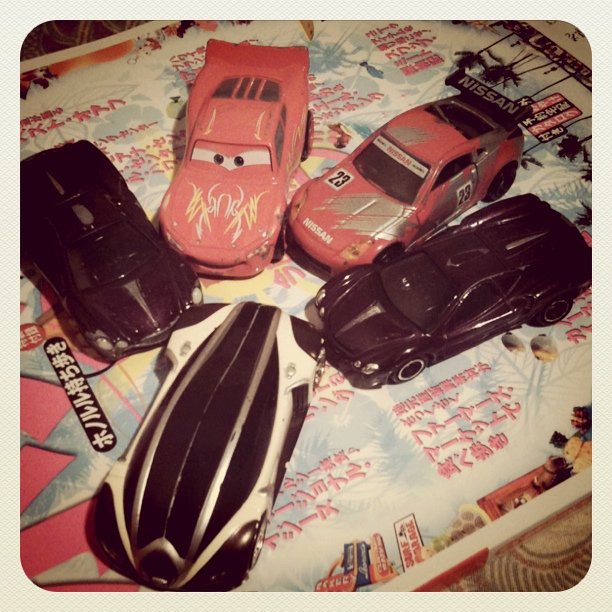This is a close-up, vintage Polaroid-style photograph depicting five matchbox toy cars arranged in a circular pattern, all front ends pointing towards the center. The cars rest on a placemat featuring Japanese text, providing a bright background primarily in white and light blue with intricate designs. Among the toy cars, two are iconic red models: one is the recognizable Lightning McQueen character from the "Cars" movie with expressive eyes on its windshield, white and yellow details on its hood, and distinctive red paint. Adjacent to it, the red Nissan Rally Car, marked with the number 23 and featuring a spoiler, stands out with gold accents. Flanking these red cars are three black cars. The one to the left displays chic white edges and silver dots with light gray stripes running across its body. The car at the top left showcases a sleek design with white and gray stripes. The vehicle at the bottom right completes the circular setup with its glossy black finish. The futuristic design, fine details, and vibrant colors of the cars contrast sharply with the intricate Asian text of the placemat, making the scene both dynamic and visually appealing.